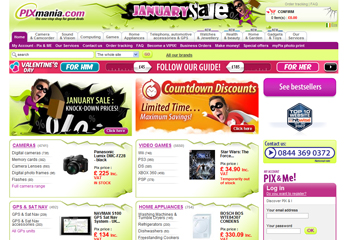The image is a bright and colorful advertisement for a discount website, likely promoting a January sale by PIXmania.com. The background is predominantly white, featuring an array of vivid colors such as red, purple, and green. In the upper left corner, set against a blue and bright green gradient, the text "PIXmania.com January Sale" is prominently displayed. Below the text, a superhero character wearing a black mask and cape is illustrated, conveying a sense of excitement and action.

A navigation bar stretches across the top of the image, showcasing various clickable categories. The 'Home' category, located on the far left, appears to be selected. The image is divided into sections, with one prominently labeled "Valentine's Day for Him." This section features various boxed items for sale, including a camera, a black frame with unspecified contents, video games, and home appliances.

Adjacent to the 'Valentine's Day for Him' section is a similar segment labeled "For Her," indicating other clickable shopping categories tailored for different audiences. Additionally, there is an eye-catching "Bestsellers" section highlighted in pink, which users can click on to explore popular items.

In the bottom right corner, a small box reads "PIX & Me," likely referring to a personalized section or account feature on the website. Nearby, a login area is present, inviting users with existing accounts to sign in.

Overall, the image vibrantly showcases the diverse product offerings of PIXmania.com, promoting their January sale with lively colors and dynamic design elements.